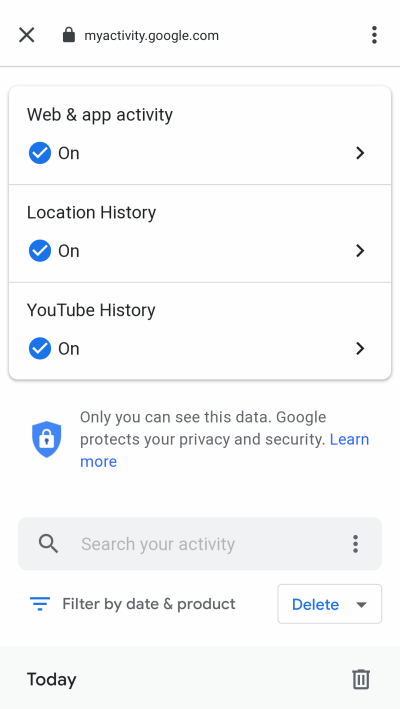The image displays a phone screen showcasing the "myactivity.google.com" webpage. At the top, the URL "myactivity.google.com" is visible, with a small 'X' icon to the left for closing and a three-dot ellipsis to the right, likely for accessing settings. 

Below the URL, there's a segmented box divided into three sections:

1. **Web & App Activity** - Indicated by a blue circle with a white checkmark, marked as "On," with an arrow suggesting it can be edited.
2. **Location History** - Similarly marked as "On" with a blue circle and white checkmark, accompanied by an arrow for editing.
3. **YouTube History** - Also turned "On," featuring the same blue circle and white checkmark with an editing arrow.

Following these sections, there's a blue shield icon with a white lock, followed by a message stating, "Only you can see this data. Google protects your privacy and security." A blue hyperlink labeled "Learn more" is available for additional information.

Further down, a search bar prompts users to "search your activity." Beneath the search bar, options are displayed to "filter by date and product" with a drop-down menu and the word "delete" highlighted in blue text. Lastly, the page displays "Today" alongside a garbage can icon, implying the ability to delete today's history entries. This interface allows users to update and manage their browsing history and activity on Google services.